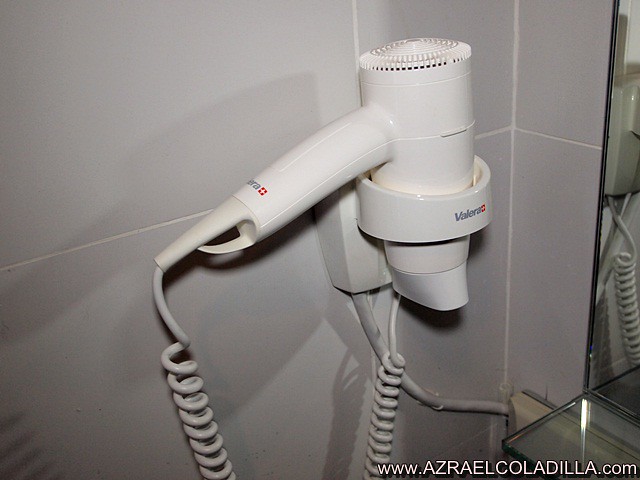The photograph depicts the interior of what seems to be a hotel room, featuring a hair dryer prominently placed in the center. This white hair dryer, branded with the name "Valera" in gray and red text, is mounted on the wall inside a specially designed holder. The holder and dryer are connected by a long, coiled cord resembling a corkscrew. The wall behind the hair dryer consists of large, off-white or light gray tiles, providing a clean and modern backdrop. To the right, a mirror is partially visible, reflecting parts of the hair dryer. At the bottom right corner of the image, the website www.azraelkoledia.com is displayed in white text.